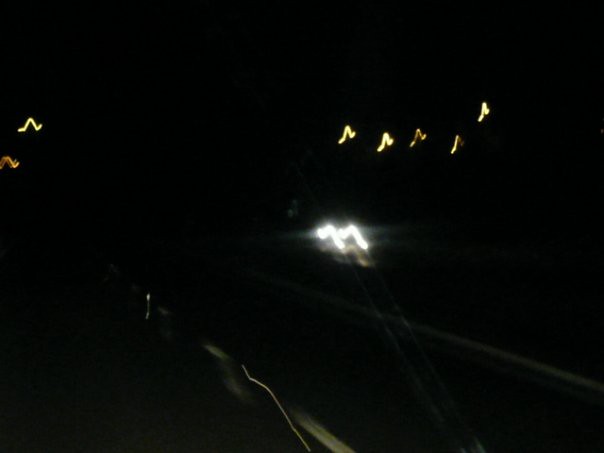This image depicts a blurry nighttime scene of an asphalt road, likely taken from a moving car. The overall background is nearly pitch black, emphasizing the darkness of the setting. At the center of the image is the road with a white-dotted centerline, illuminated by various blurred lights. To the lower part of the image, there are two beams of light seemingly emanating from the headlights of an oncoming vehicle, creating a glare effect. To the left and far right of the road, there are squiggly lines and streaks of light in hues of yellow and gold, possibly streetlights or reflections, resembling upside-down 'V' shapes. The texture on both sides of the road suggests the presence of grass, with the robust darkness continuing outwards, enveloping the entire scene.